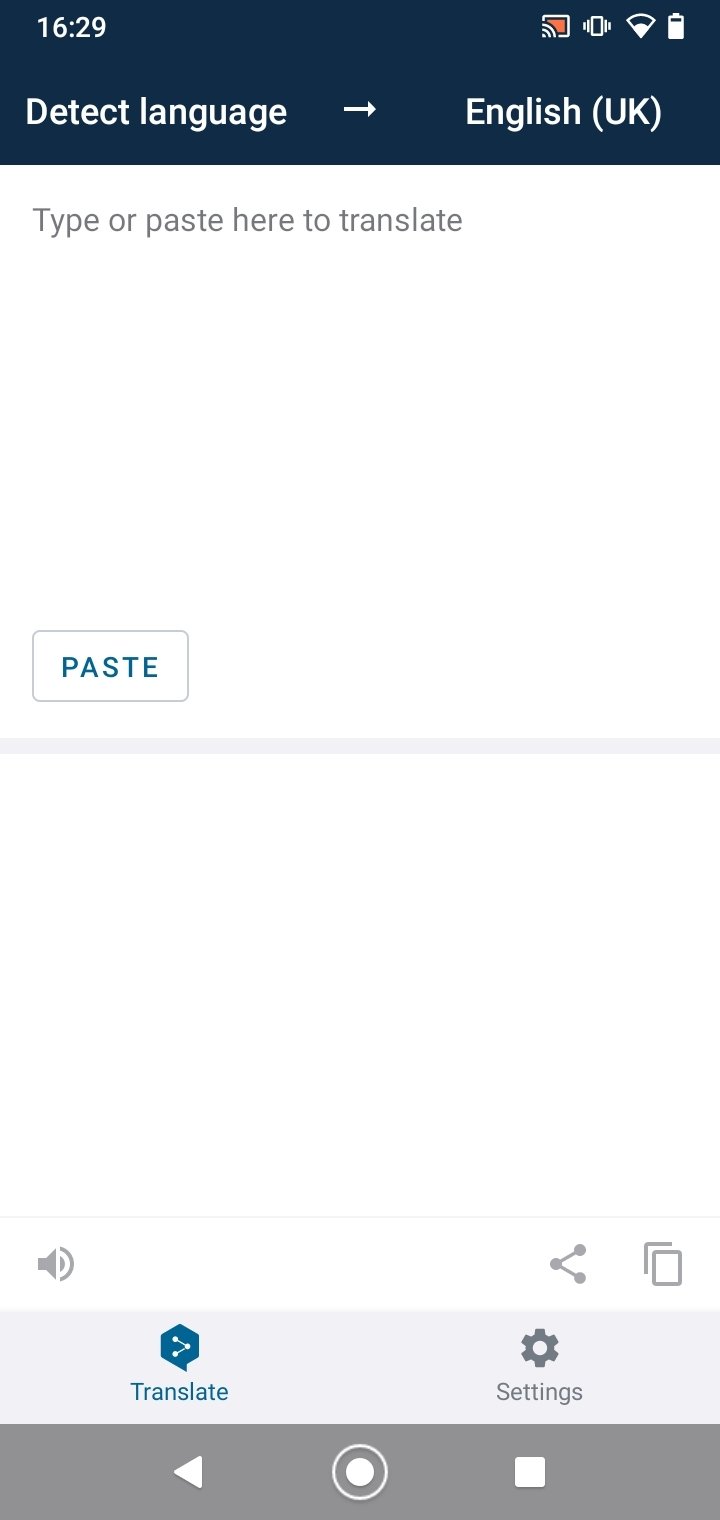This image displays a smartphone screen featuring a translation app interface. At the top, a thick navy blue banner spans across the screen, showing the current time "16:29" in white text on the upper left corner. To the right, near a nearly full battery icon, are various other status icons whose functions are not specified. Below the banner, the text "Detect language" with a right-pointing arrow is prominently displayed in white. Adjacent to it, the text "English (UK)" is visible.

The main body of the screen has a white background with a gray text prompt stating, "Type or paste here to translate," followed by an empty white space intended for user input. At the bottom of this section, a button with a gray border is labeled "Paste" in bright blue text. Flanking this button, there is a gray speaker icon on the left for audio input and a share icon on the right for sharing options.

Further down, a light blue background houses a bright blue highlighted "Translate" button. To its right is a settings icon paired with the word "Settings." Finally, at the very bottom of the screen is a dark gray banner containing main navigation buttons: a centrally located home button, a back arrow on the left, and a square button on the right.